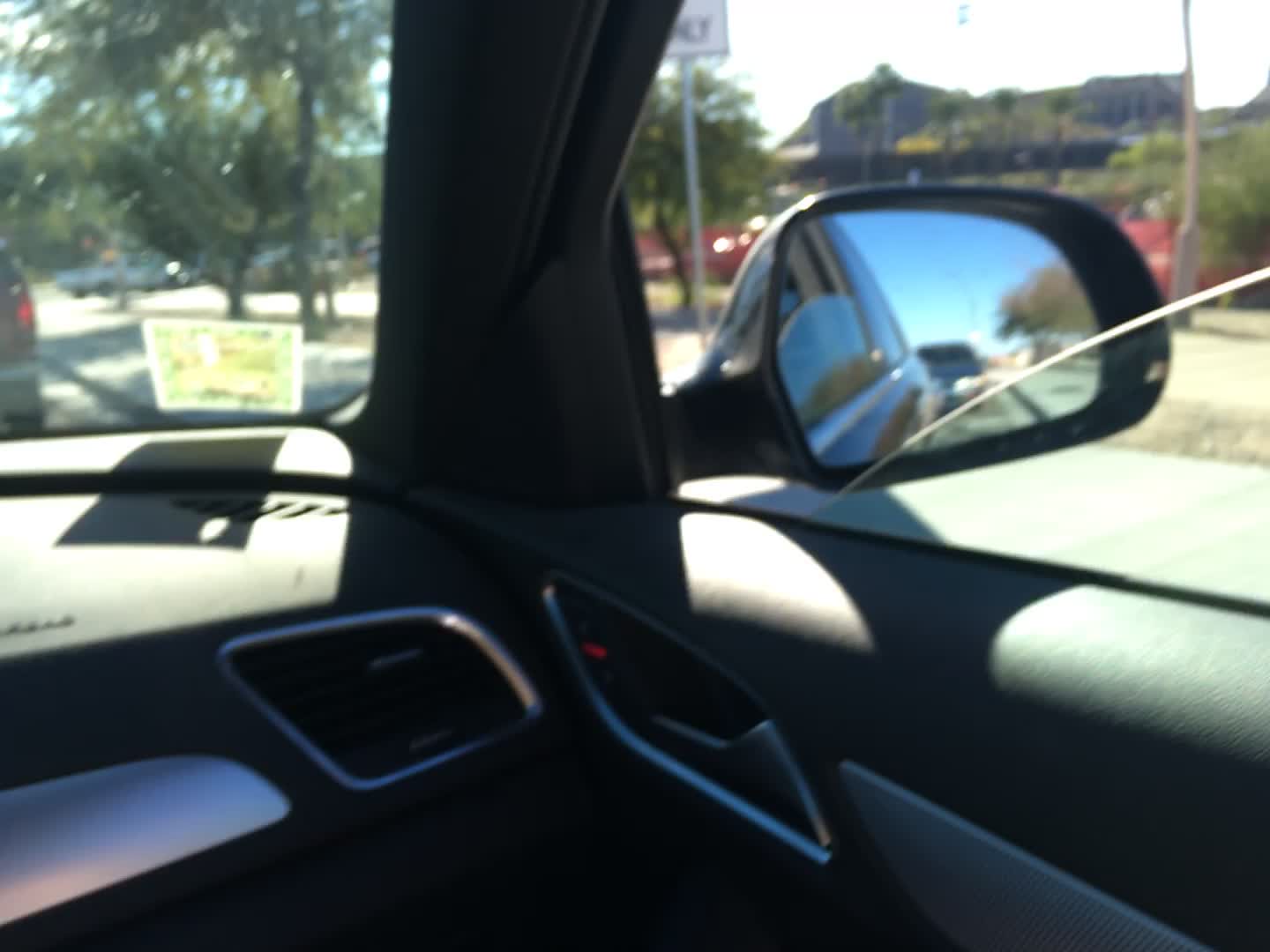This photograph, taken from the passenger seat of a dark gray or black vehicle, captures a detailed and slightly blurry scene through the windshield and partially rolled-down side window. The image includes an interior view showing the car’s door handle, dashboard, and a vent. The black rearview mirror, positioned on the right, reflects a back window that is halfway down, revealing a darker-colored car behind with its headlights on, suggesting a daytime setting. The windshield displays a yellow toll road marker or similar decal. Outside, the photo frames a busy scene with a tree to the right of the car ahead, a grey and white street sign, additional trees, and a large indistinct building in the background. Red objects and a white sky further blur the exterior, adding to the complexity of the image.